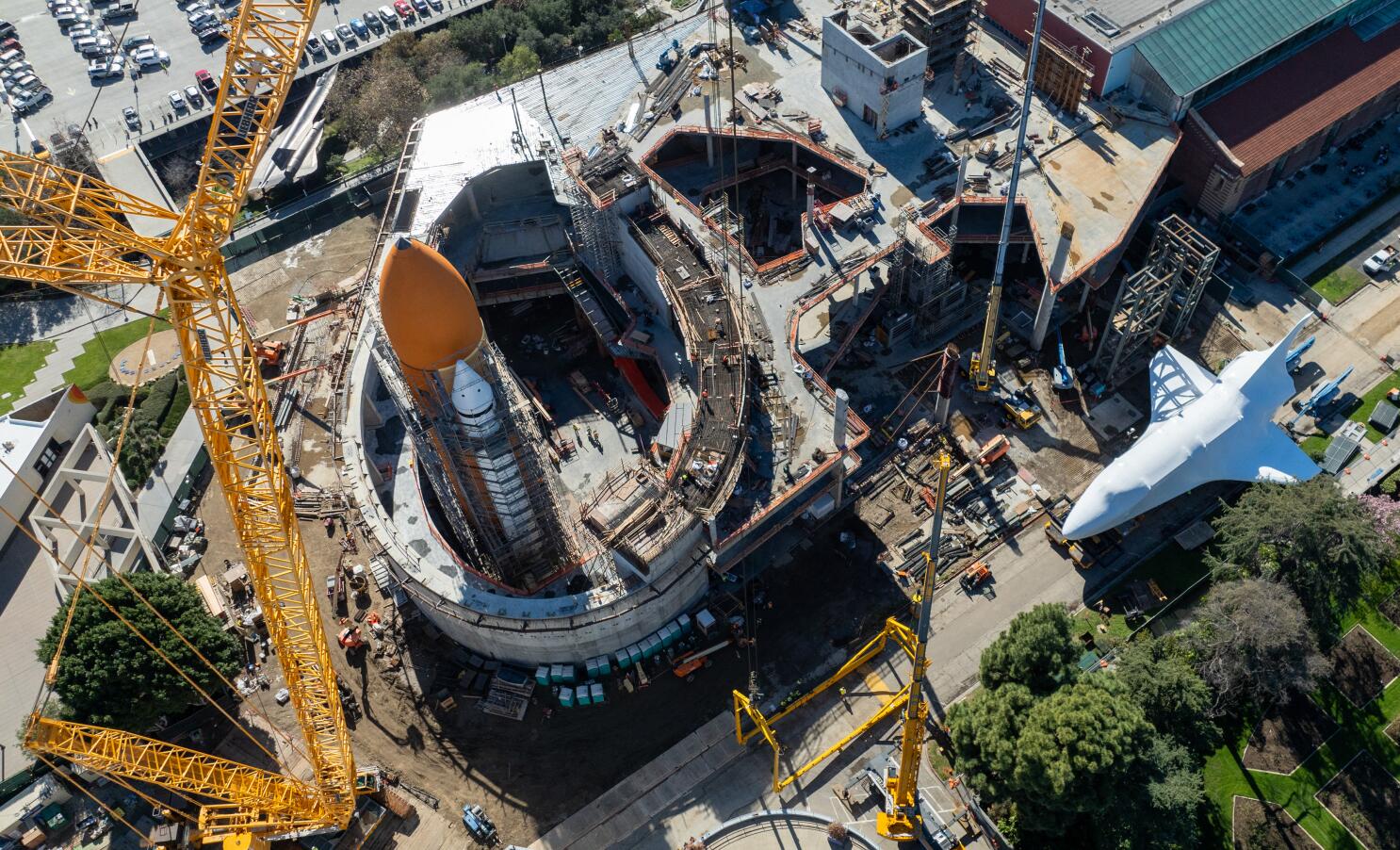This aerial image depicts a bustling industrial facility, likely a rocket manufacturing or launch site, filled with numerous ongoing construction activities. Central to the scene is a prominent orange rocket, adorned with white miniature rockets attached to its sides. It appears to be positioned within an open-air, stadium-like structure, surrounded by numerous workers and an array of construction materials. Adjacent to this scene is a large, yellow crane extending above a partly dilapidated yet substantial building, emphasizing the continuous development within the facility.

To the left, a spacious parking lot teems with parked vehicles, indicating the presence of many personnel on-site. Meanwhile, the top right of the image reveals a stationary white plane or shuttle, adding to the aerospace theme of the facility. The terrain is a mix of dirt and concrete, interspersed with patches of trees and grassy areas, though predominantly industrial in character. The setting is bathed in daylight, with clear evidence of meticulous upkeep in certain green patches. While the exact location remains ambiguous, the detailed view suggests a significant, industrious enterprise at work.